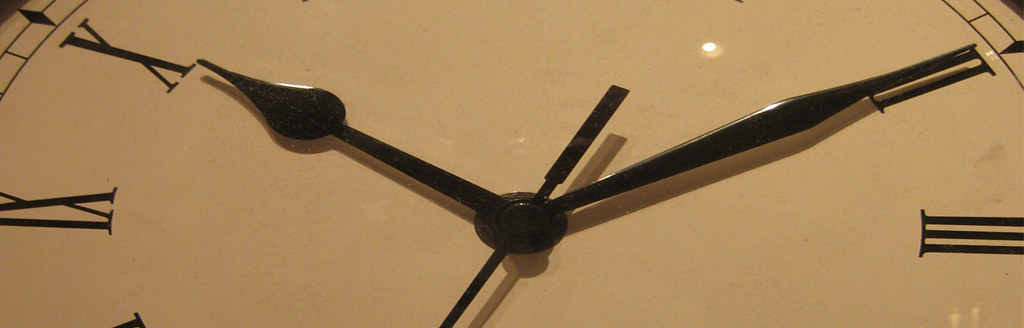This image showcases a close-up view of a large clock face. The clock features a light beige background that contrasts with bold black Roman numerals marking the hours. In the center are two prominent black hands with teardrop-shaped pointers and a slender second hand, all casting subtle shadows onto the clock face. Just above the larger hand, there is a tiny dot of white light, possibly reflecting from the polished surface of the clock. Visible in the frame are the numerals III (3), IX (9), and X (10), indicating the classical design. The detailed craftsmanship of the clock highlights its elegance and timeless appeal.